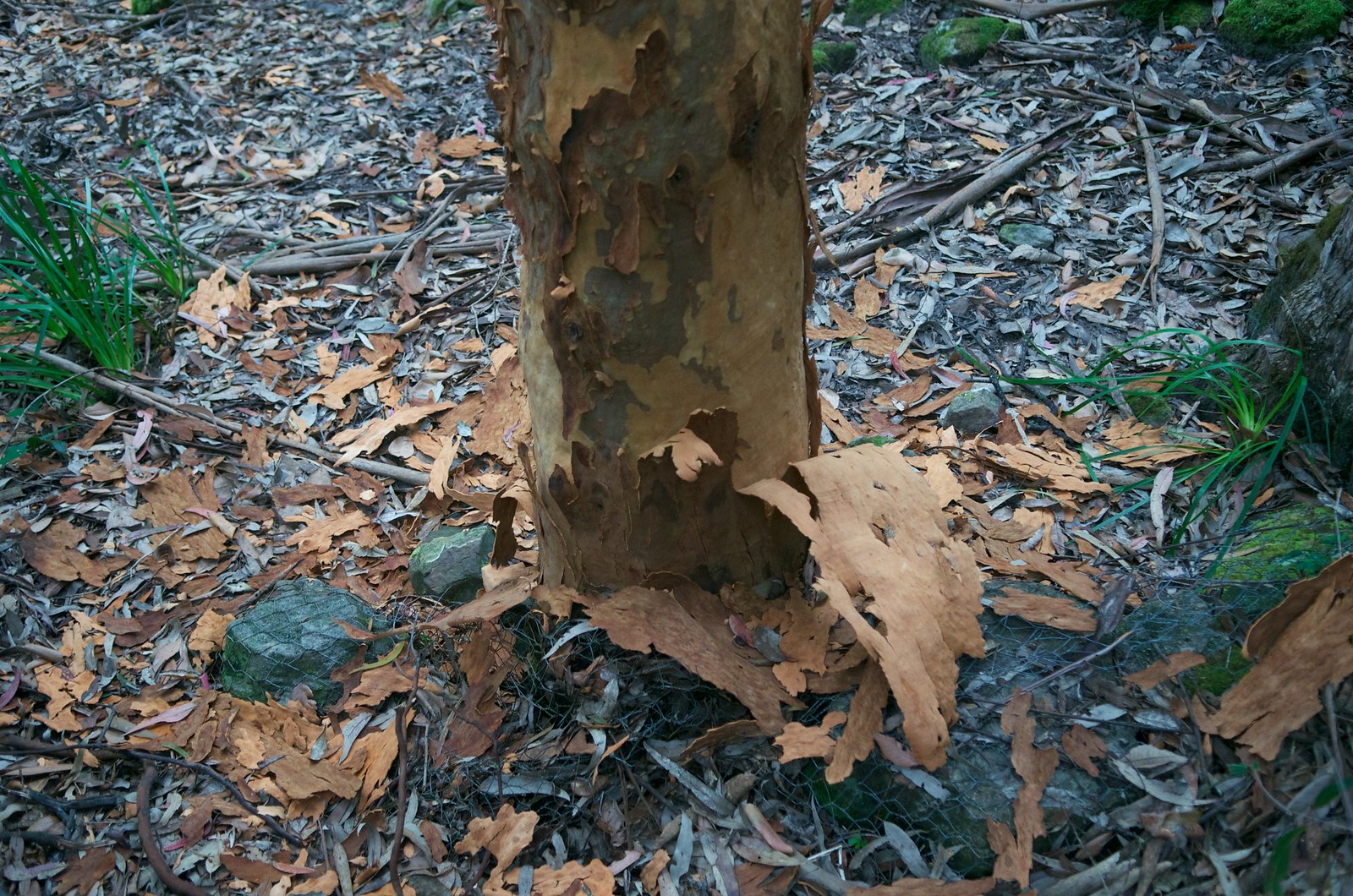The photograph, rectangular in shape and taken outdoors in a forest-like setting, captures the base of a tree where the bark is peeling off in multiple, thin layers. The light in the image is bright and natural, casting a neutral ambiance rather than a warm, yellowish glow. The ground is littered with old leaves, twigs, and various-sized rocks scattered around. Notably, several pieces of peeled bark have fallen and now lay dispersed around the tree's base. Sprigs of green grass-like plants sporadically punctuate the mostly barren ground. Large branches and sticks are also visible, along with plants dotting the left, right, and top edges of the photograph, giving a sense of dense, surrounding foliage.